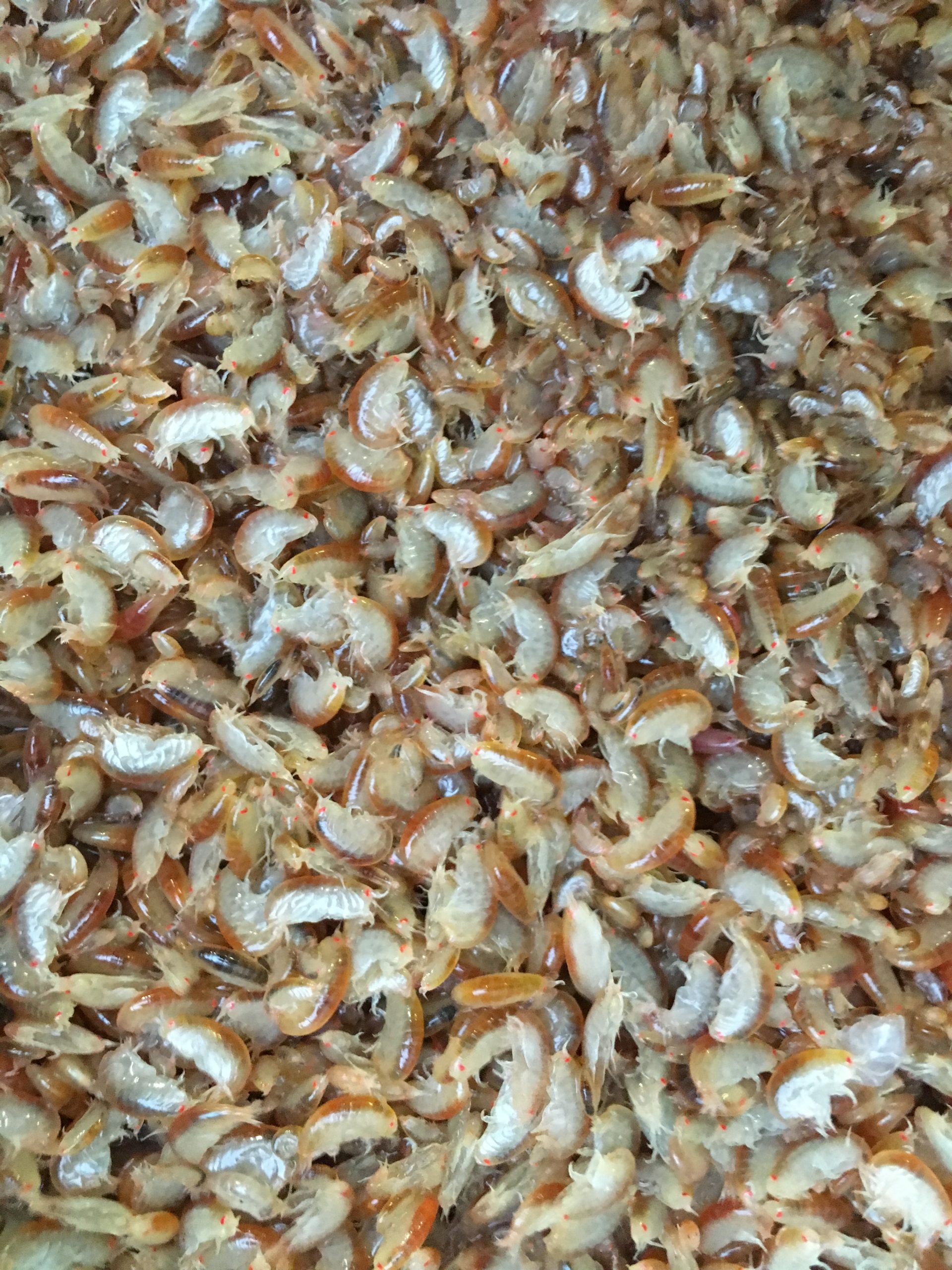The image depicts thousands of small, translucent sea creatures, resembling shrimp or krill, densely packed together, filling the entire frame. Each creature is about the size of a fingernail or smaller. Most have clear bodies with a brown tint on the dorsal side, while a few exhibit darker black coloration. The scene is brightly lit with natural light reflecting off their wet, segmented bodies. They vary in orientation, with some stretched out and others curled. This close-up, detailed photograph shows no other objects or animals, emphasizing the mass of these crustaceans, likely captured from a net.